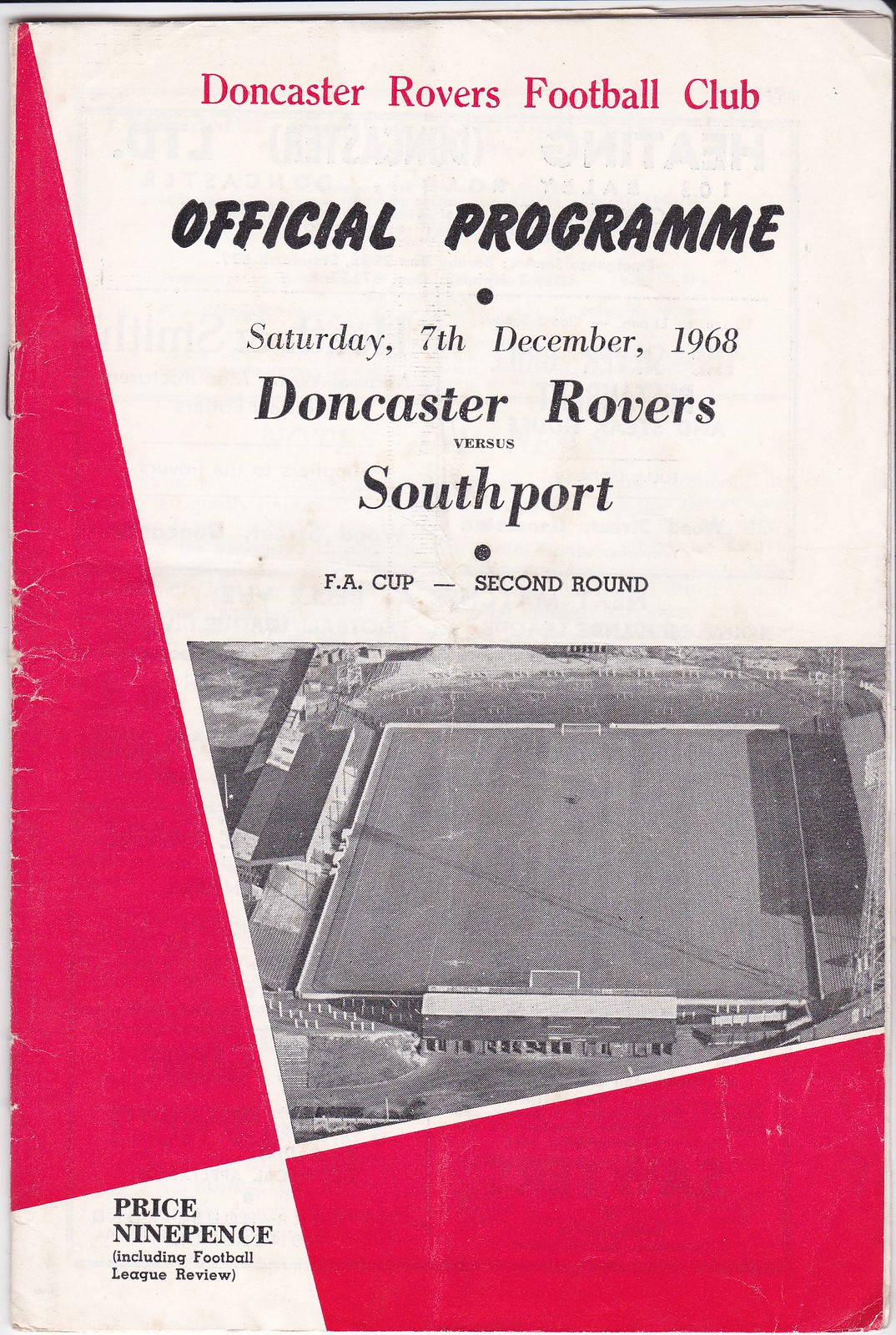The image displays the front page of an official program for the Doncaster Rovers Football Club, styled like a vintage magazine cover with a mostly white background accented by geometric red and pink shapes. At the top, "Doncaster Rovers Football Club" is prominently printed in red letters, followed by black lettering that reads "Official Program, Saturday 7th, December 1968, Doncaster Rovers versus Southport, FA Cup Second Round." An overhead black-and-white photograph of an empty football stadium is prominently featured in the center. Surrounding the photo, on the left side runs an elongated pink triangle, accompanied by a rectangular pink shape near the lower portion, adding a vibrant contrast. In the lower left corner, the price "nine pence" is indicated, including a "Football League Review." The program appears slightly worn, with visible staples suggesting it has been handled.